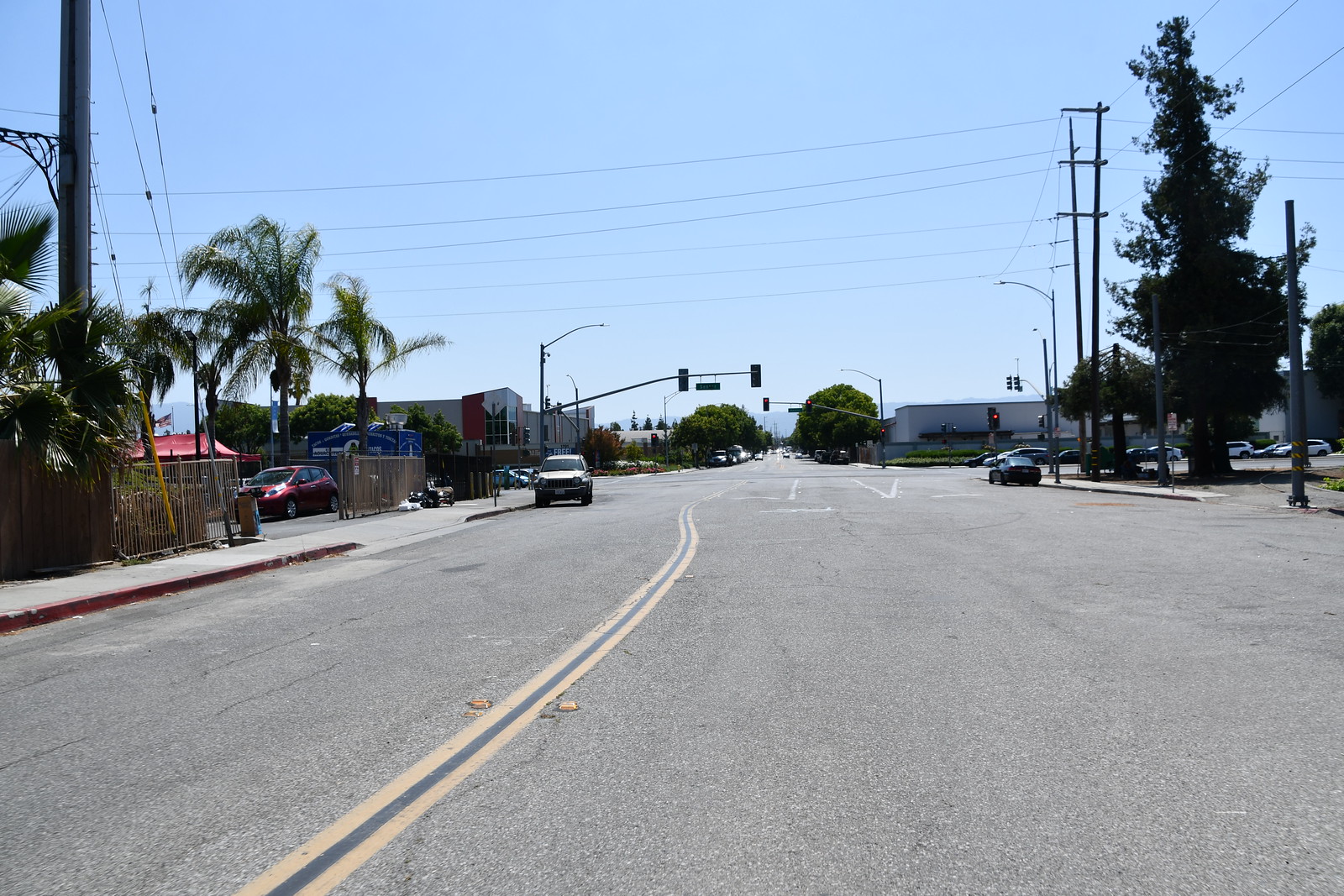The image showcases a bustling intersection in a small town under a clear, blue sky. The road features three lanes, with two lanes dedicated to oncoming traffic from the left and three lanes on the right side for traffic heading in different directions: left, right, and straight. A car on the right side is turning right, while an oncoming car approaches the photographer from the left side.

On the left side of the road, several palm trees add a tropical touch, and a hotel can be seen further down. The right side of the road is lined with regular trees, a warehouse-like building, and a cabana-style structure with more palm trees. Electricity poles and wires span across the scene, contributing to the town's infrastructure.

The colors in the image are vivid and varied: the black asphalt is divided by a prominent yellow strip marking the lanes, red cars add bright spots of color, green trees bring life to the surroundings, and the brilliant blue sky stretches overhead.